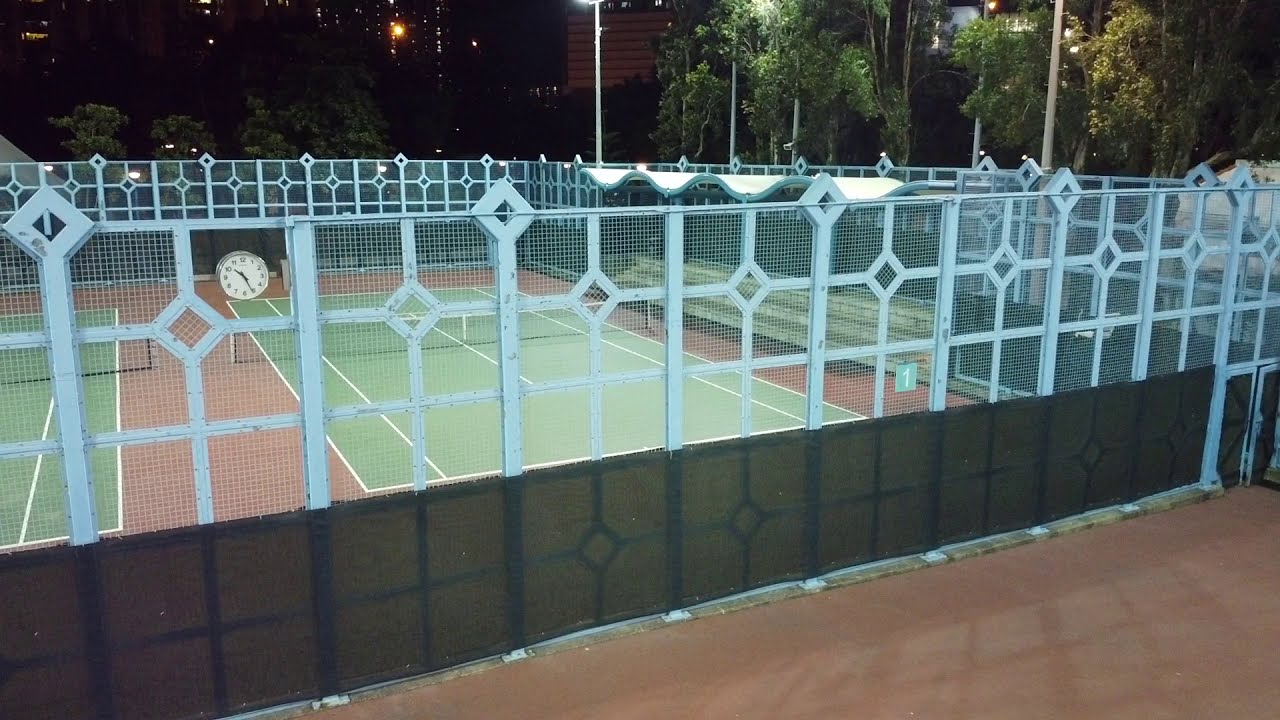This image, taken from an elevated perspective, showcases a pair of illuminated public tennis courts set against a twilight or nighttime backdrop. The courts, marked with the typical green surface and white lines, are enclosed by tall, decorative fencing characterized by bluish-gray steel grid patterns and mesh, along with wider gray bars and decorative elements resembling window panes and diamonds. The fencing is more elaborate than typical chain link, suggesting a more upscale or carefully designed environment. Between and around the courts, the ground features a reddish-orange surface. Notably, there's a clock mounted on the fence, visible against the backdrop of trees and bushes, indicating it could be part of a larger park or forested area. Tall light towers are strategically placed to illuminate the courts. A green sign labeled "Court One" can be seen, along with some possible bleachers on one side, which add to the setting's detail and functionality.